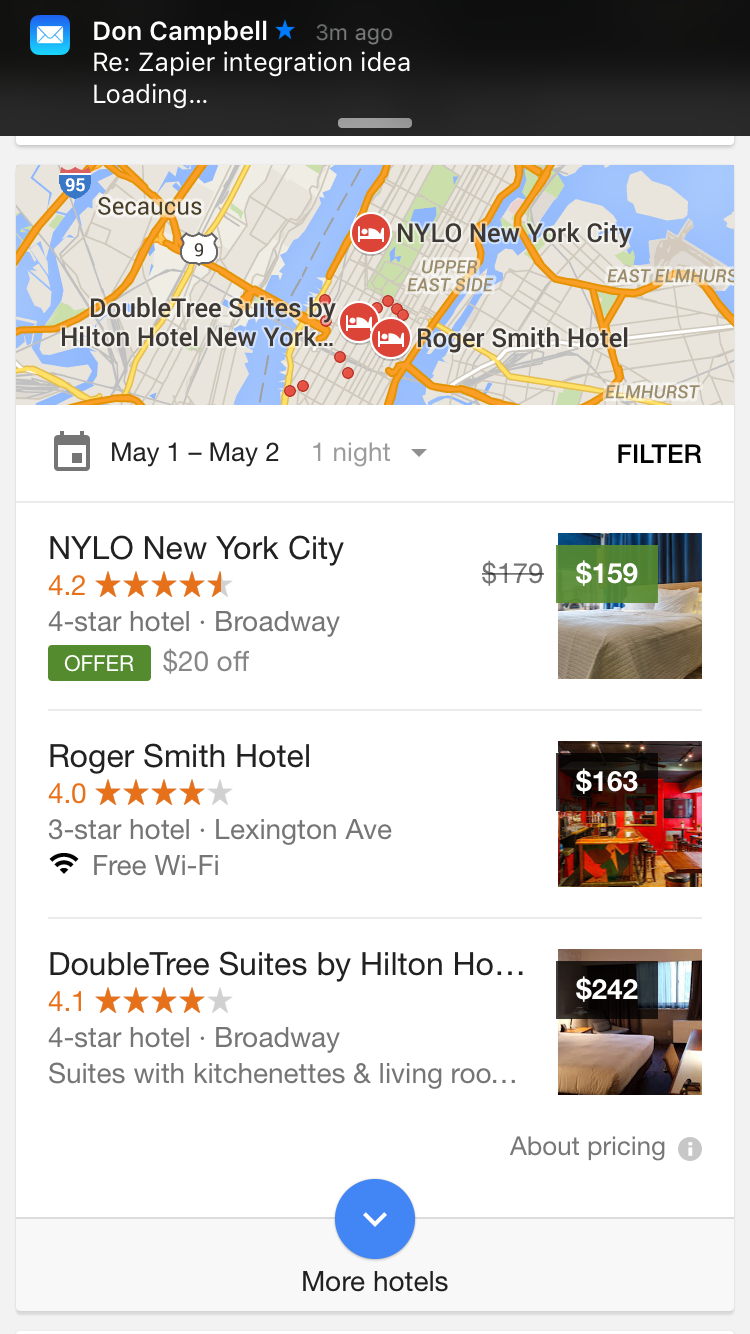A screen capture of a mobile web application interface displaying hotel options in lower Manhattan. In the upper left corner of the image, the name "Don Campbell" is visible, accompanied by a blue star, with "3M Ago" written to the right indicating the time since an interaction. Below this, there is a notification titled "RE: ZAPIER integration idea," followed by a "loading" message.

The primary section of the screen showcases a map of part of Manhattan, identified by several icons resembling people sleeping in beds, likely indicating hotel locations. Below the map, a list of hotels is presented, beginning with "NYLO New York City," a four-star hotel with a rating of 4.2 stars. It offers a special promotion of $20 off, displaying a photo of a bed with a green overlay indicating a price of $159.

The next hotel listed is the "Roger Smith Hotel," rated 4.0 stars and categorized as a three-star establishment. Located on Lexington Avenue, it offers free Wi-Fi and is priced at $163.

Lastly, the "DoubleTree Suites by Hilton" offers four-star accommodations with a 4.1-star rating. Situated on Broadway, this hotel features suites with kitchenettes and living rooms, priced at $242.

This app appears to be helping the user search for hotels in lower Manhattan, providing detailed descriptions, ratings, locations, amenities, and prices for each option.